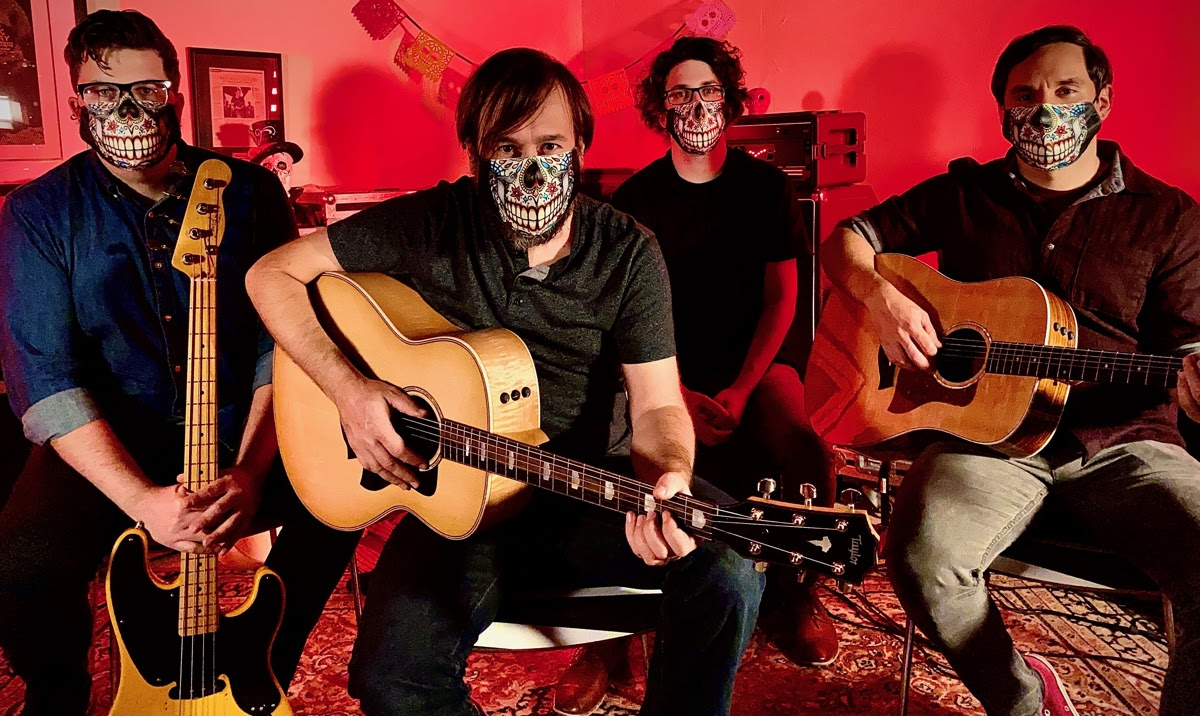The photograph captures a band consisting of four members seated with a striking red light cast over them, tinting the white wall and objects behind them in red. Starting from the left, the first person is dressed in black denim pants and a blue denim button-up shirt with sleeves rolled up to their elbows. They wear black-framed glasses and a face mask that depicts the bottom half of a skull, and they hold the neck of an electric guitar, with its body resting on the red carpet. The second person from the left is wearing a short sleeve black shirt with one button undone, paired with dark blue denim pants. He holds a light brown acoustic guitar. The third person, dressed similarly in dark blue denim pants and a collared shirt, does not have a guitar. The last person on the right also wears dark blue denim pants affected by the red lighting and holds an acoustic guitar. Notably, three members are wearing face masks designed with a skull motif, enhancing their thematic look. Behind them, the wall features various pictures and news articles, and equipment such as a carrying case and a trunk is visible amidst the red backdrop. Additionally, a decorative skull with a hat is noticeable behind the leftmost member. The overall composition of the image suggests a band set up for a performance, enhanced by their casual yet coordinated attire and the dramatic red lighting.